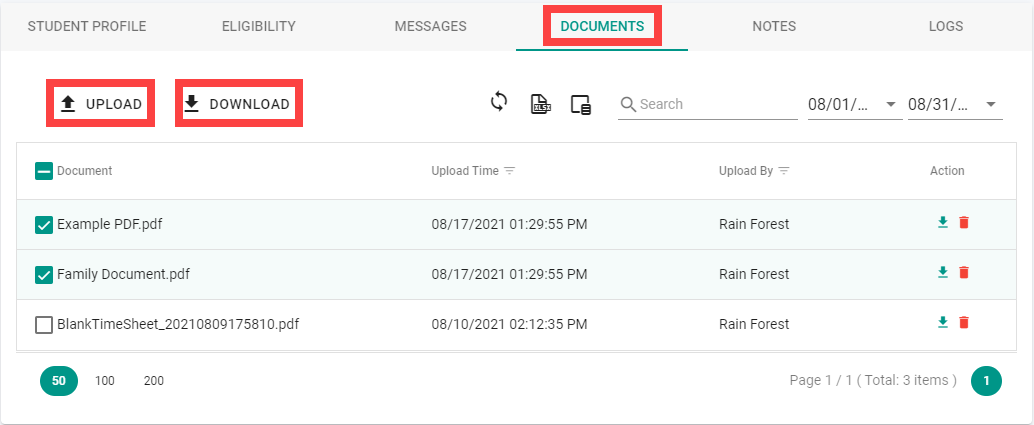In this computer-generated image, the background is a pristine white, providing a clean and clear canvas for the structured elements displayed. At the top, there is a horizontal navigation bar with segmented labels: "Student Profile," "Eligibility," "Messages," "Documents" (which is highlighted with a thick red border, indicating it is the active tab), "Notes," and "Logs." Below this navigation bar, there are functional icons for uploading and downloading, each accompanied by arrows pointing up and down respectively, both encased in red borders for emphasis.

Adjacent to these icons, there is a search bar designated for filtering content, followed by date selection options to refine the displayed data based on specified time frames. 

The main content area beneath these tools is organized as a table with the headers: "Document," "Upload Time," "Uploaded By," and "Action." Each row itemizes specific documents, such as "Example PDF," "Family Document," and "Blank Timesheet." For each document listed, the upload time and date are provided, alongside the identifier "Uploaded By Rainforest," indicating the user or entity that performed the upload. The "Action" column likely contains the actions available for each document, although this detail is not explicitly described.